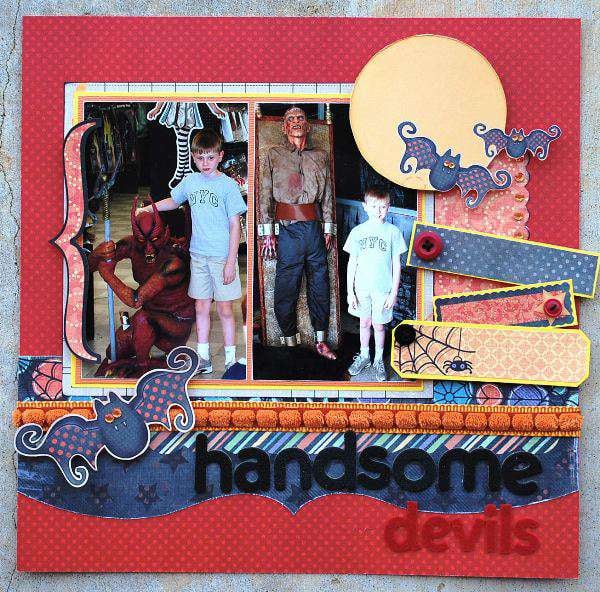This image showcases a handmade Halloween collage set against a speckled gray, orange, and brown stone-like background. Dominating the scene is a large red poster board decorated with pink polka dots, which obscures most of the backdrop. There are two main photographs nestled within the upper portion of the red poster board. In the left photo, an older little boy, dressed in an NYC short-sleeve shirt, khaki shorts, white socks, and gray tennis shoes, stands beside a menacing figure dressed as a devil. The devil, adorned in red and black with prominent horns, is kneeling and flexing its muscles with its fists together. In the right photo, a younger boy, donning the same outfit and smiling broadly, stands next to a zombie. This ghastly figure, with dark pants, blood-stained feet and face, and a long-sleeve brown shirt, appears to be strapped to a board with silver straps around its wrists. The scene is further embellished with playful cutout shapes, including images of bats, a moon, and small rectangular shapes with buttons. The bottom of the collage prominently features the phrase "Handsome Devils," with "Handsome" in black letters and "Devils" in red, creating a fittingly spooky yet affectionate tribute to the Halloween festivities.